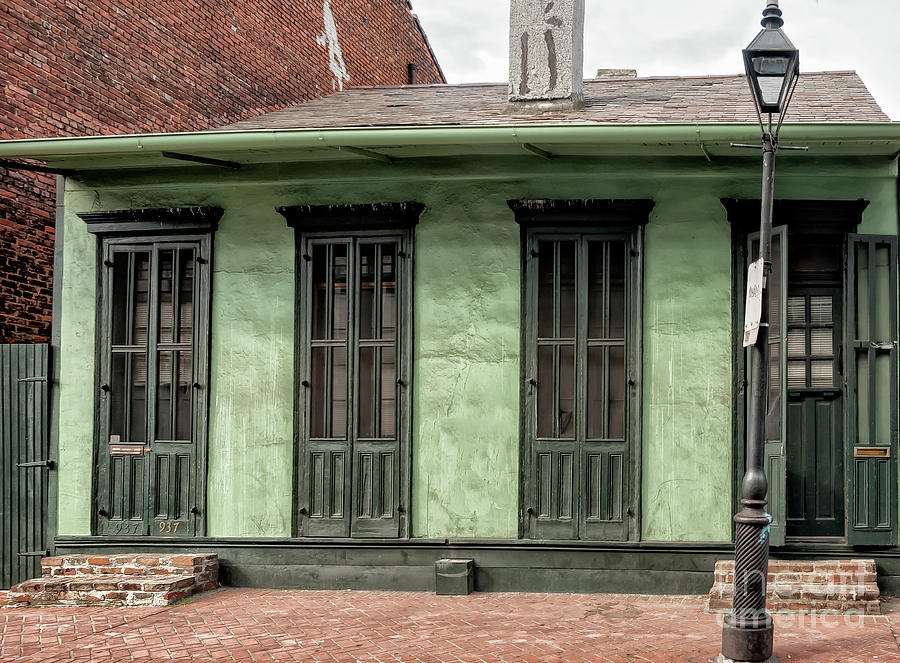The image depicts the facade of a small office building attached to a larger red brick structure. The office is characterized by its uneven green stucco walls and four tall, dark green-trimmed doors which nearly reach the top of the building. The lighter green roof forms an awning that extends about three feet over the entrance, creating a small porch area supported by two brick steps. A closer look reveals a brass mail slot on the left door, which also features the address "937." Meanwhile, the right door bears a nameplate. Two identical windows, matching the size, shape, and color of the doors, are situated between the entrances. The front area is paved with red bricks, complementing the brick steps. Additional details include a dark green vertical slatted wood fence on the left-hand side, a streetlight with a white sign positioned in front of the building, and a white chimney atop the adjacent brick structure.